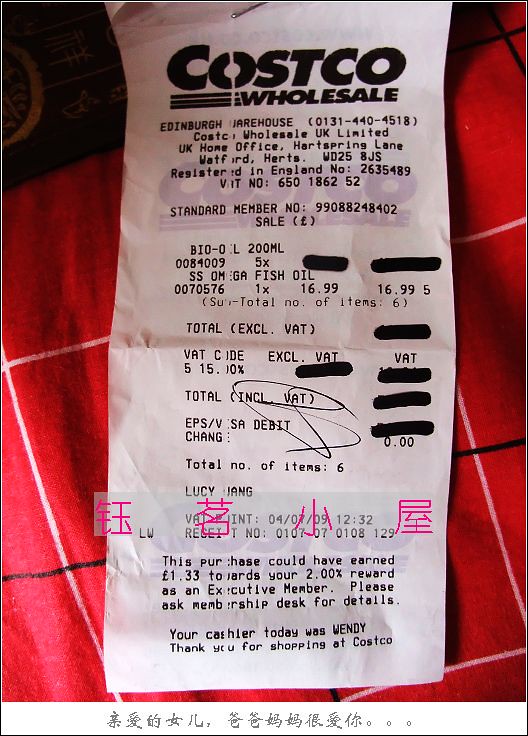In the image, a textured background of vibrant red fabric adorned with white and black stripes creates a striking checkerboard effect. Placed centrally on the fabric is a slightly worn and bent white receipt, oriented vertically. In crisp black ink at the top, the receipt details read: "Costco Wholesale, Edinburgh Warehouse, Costco Wholesale U.K. Limited, U.K. Home Office, Waterford Heart," followed by the registration information in England. It mentions the standard member number as 99088248402. Listed on the receipt is a single item, "SS Omega Fish Oil," priced at $16.99. At the bottom, the receipt identifies Lucy Yang as the recipient and notes, "Your cashier today was Wendy. Thank you for shopping at Costco."